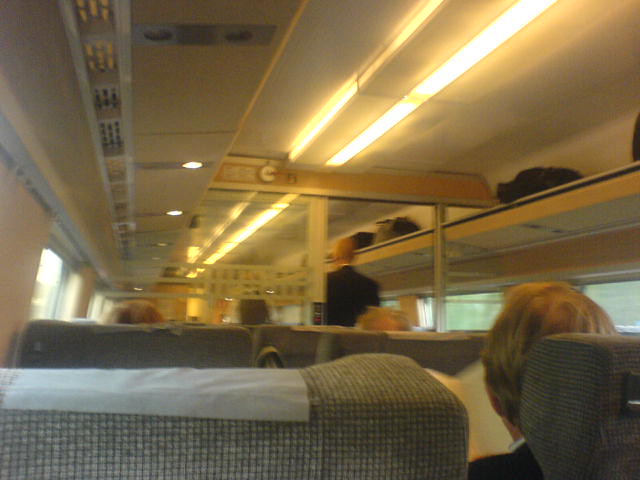This image captures the interior of a train from the perspective of someone sitting in a window seat on the left side. Directly in front is the back of the seat, featuring a gray cushion with a black mesh pocket at the top and a light gray headrest cover. While this seat is unoccupied, there is a person sitting in the seat diagonally in front to the right. The ceiling of the train is fitted with long track lighting running the length of the walkway, and individual reading lights positioned above each seat.

A few aisles ahead, a man in a black suit jacket and white shirt is standing and walking away. The train appears sparsely populated, with a few passengers scattered throughout the seats. Overhead compartments contain luggage and bags, and a sign with blurred lettering is mounted on poles extending up to the ceiling. The image also captures the tops of a few passengers' heads, including a gray-haired individual and another bald man in black attire, possibly suggesting a formal or business context.